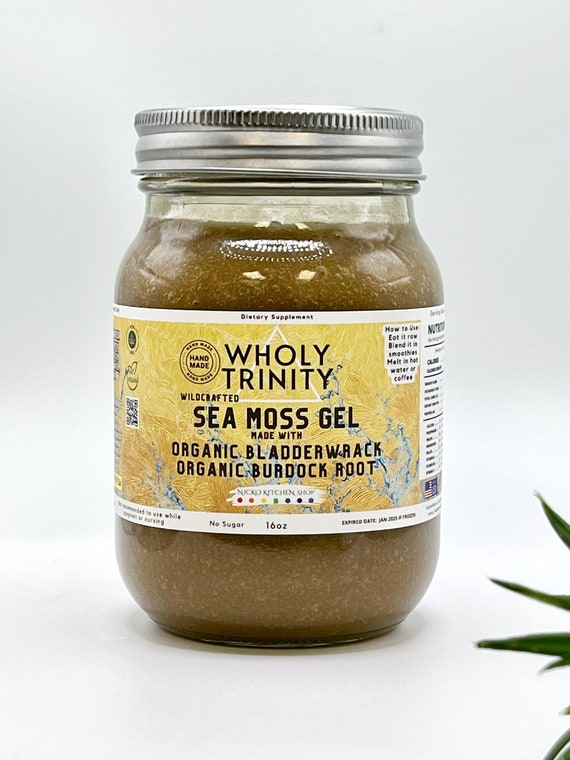The photograph before me is a vertically-oriented, full-color image of a small mason jar containing a green, textured sea moss gel. The clear glass jar features a silver twist-on lid and bears a green label with black print. The label prominently displays the brand name "Holy Trinity" along with the product description: "Wildcrafted Sea Moss Gel with Organic Bladder Wrack and Organic Burdock Root." Additional text details on the label include instructions for use, stating "eat it raw, blend it in smoothies, melt in hot water or coffee," as well as information on the product being handmade and from "Neko Kitchen Shop." The jar is 16 ounces with no sugar added, as noted on the label. The background of the image is predominantly white, complemented by the presence of plant leaves in the lower right corner, suggesting a natural, holistic vibe. The composition and clarity of the photograph give it the appearance of an advertisement.